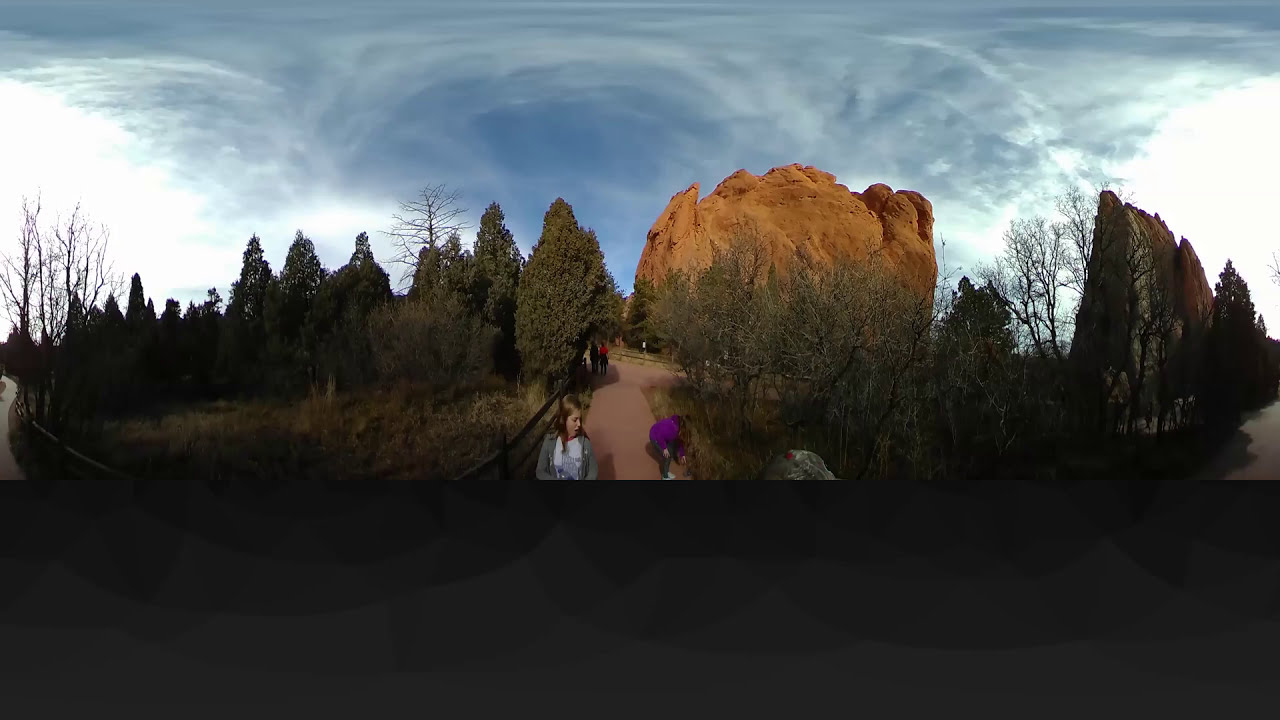In this detailed panoramic outdoor image, we see a scene dominated by a significant light brown rock formation that rises around four to six stories tall, likely a prominent tourist attraction. The top of this multi-shaped rock draws the eye, while to its right stands a triangular-shaped rock pointing towards the sky. Central to the image, a dirt or stone walkway cuts directly through the scene, where several people are visible. Most notably, a woman with brown hair, clad in a gray sweater and white shirt, walks towards the camera. To her right, a grassy area bordered by a wooden fence sits, with another woman in a purple jacket bending over into the grass. The left side of the path also features grassy areas and trees, extending towards the center alongside the walkway. Behind the main subjects, the path continues with more distant figures wandering through the scene.

The background is rich with natural elements: clusters of trees between and around the rock formations, as well as an expansive grassy terrain. The sky above is blue, dotted with patches of white clouds, suggesting a clear, sunny day ideal for outdoor exploration. Enhancing the ambience, the image bursts with a variety of colors including black, gray, green, brown, purple, red, blue, white, and orange, all contributing to the vivid portrayal of a serene nature trail. There is no text displayed in the image, keeping the focus solely on the picturesque landscape and its visitors.